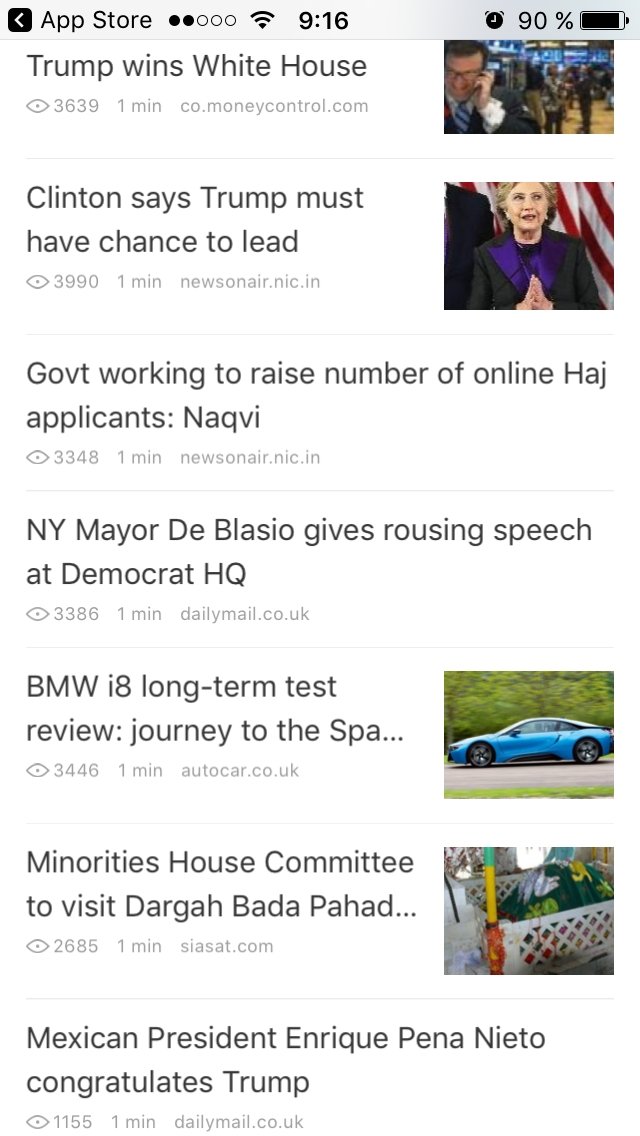The image is a screenshot featuring a collection of different news articles, showcasing only their titles and brief metadata. The first article prominently headlines "Trump Wins White House" followed by a small eye icon and the number "3639," indicating the total views or reads the article has accumulated. The second headline states "Clinton Says Trump Must Have a Chance," while the third reads "Government Working to Raise Number of Online Hajj Applicants." The fourth article title is "NY Mayor De Blasio Gives Rousing Speech at Democrat HQ." The fifth headline, "BMW i8: The Long Term Test Review," discusses the automotive model, and the sixth title, partially cut off, mentions something pertaining to a Mexican president. Each article appears succinct, with just enough information to engage readers and prompt further exploration.